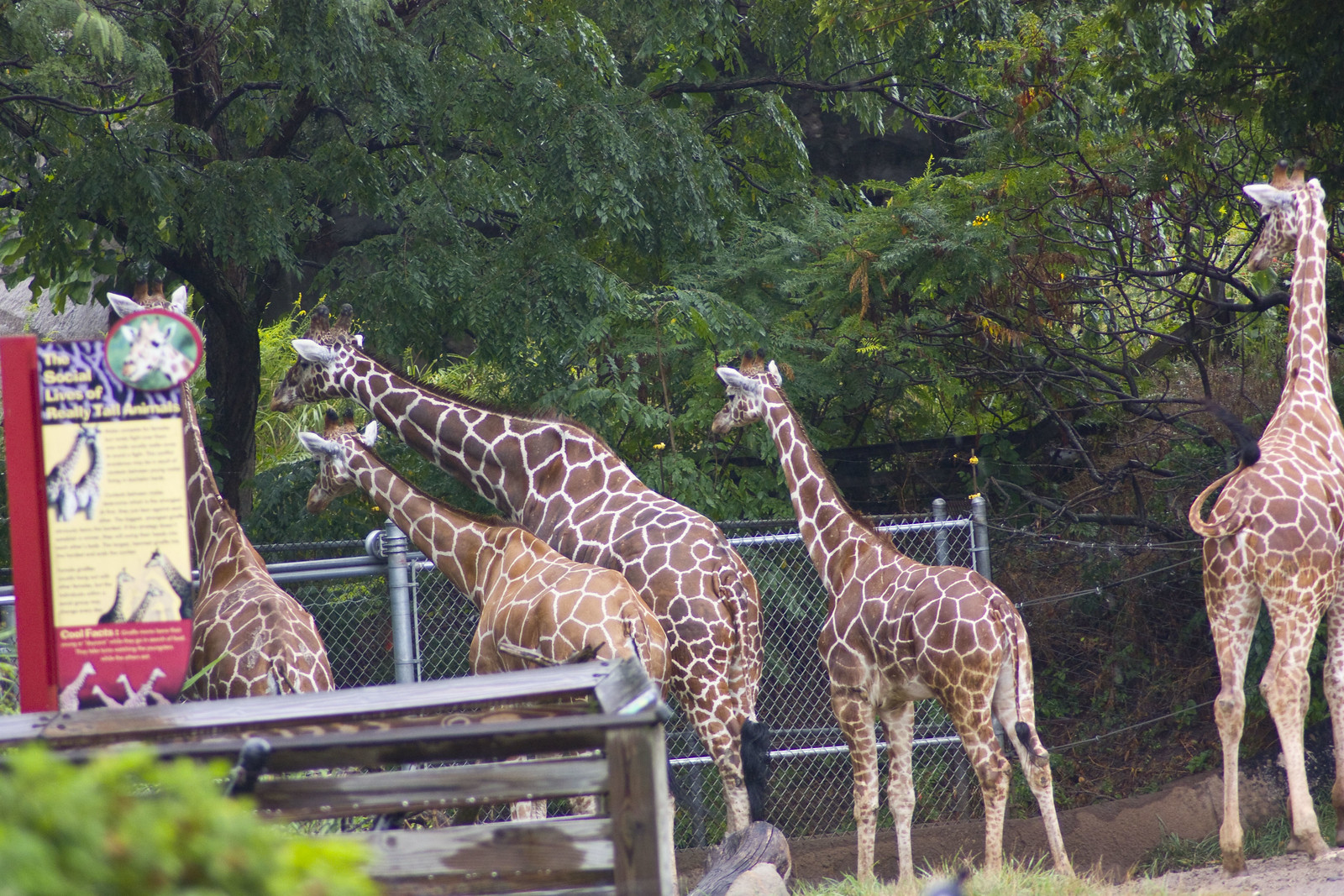The photograph is a landscape-oriented image featuring five giraffes in what appears to be a zoo or reserve. All the giraffes are facing away from the viewer, looking toward the left side of the image with keen interest, likely fixated on a zookeeper or someone preparing their food. Four giraffes are positioned closer to the left and are seen peering over a large silver chain fence, while the fifth, slightly taller giraffe stands towards the far right, similarly focused on the left. The left side of the image also features an informational post or board with facts about the giraffes, including a circled picture of a giraffe. The background is filled with numerous tall trees, their foliage displaying various shades of green interspersed with hints of brown. This dense treescape gives the impression of a forest-like environment surrounding the giraffes.